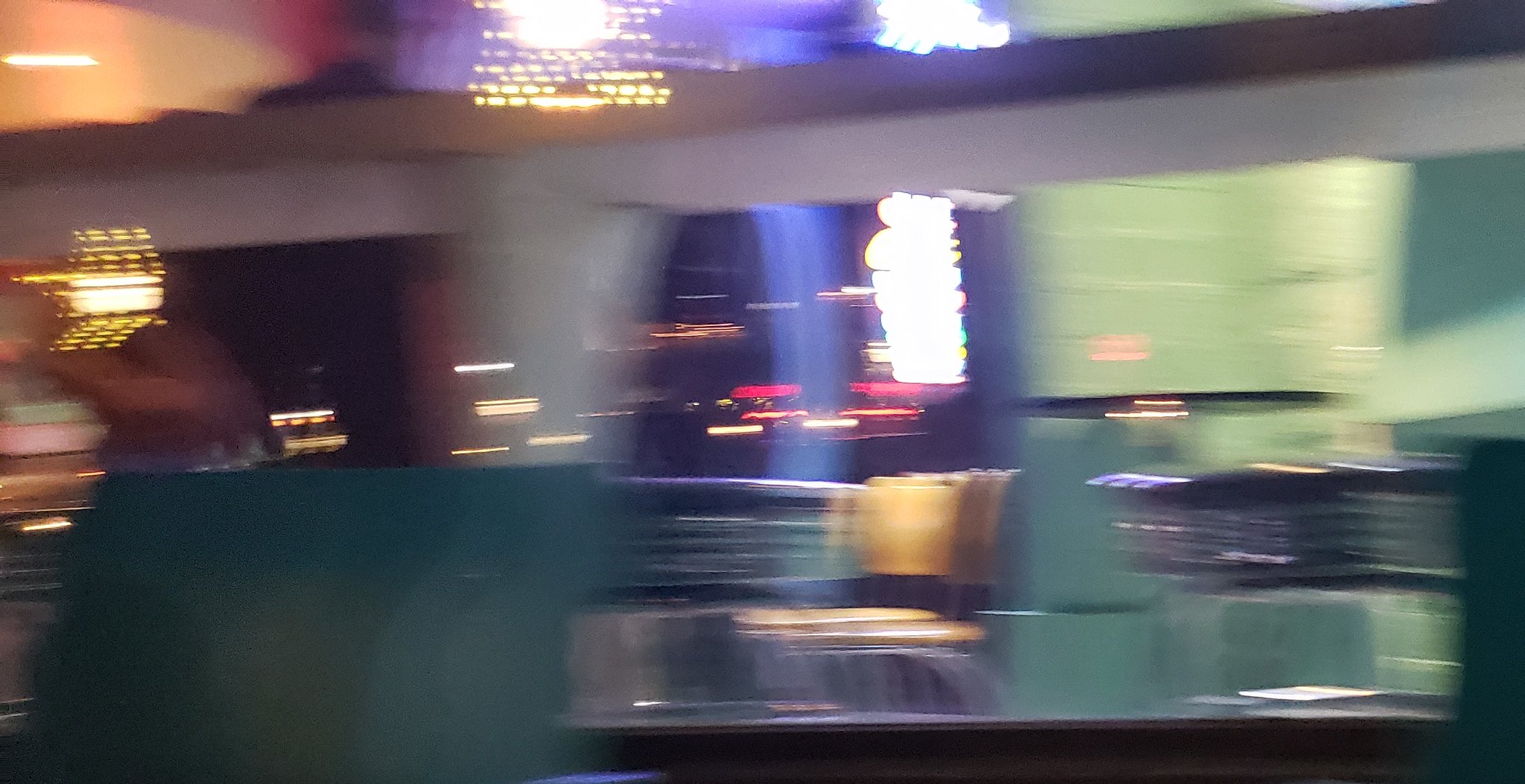This photograph appears to be taken in a restaurant or dining space at nighttime while the photographer was in motion, resulting in a significantly blurry action shot. The central focus is a small grouping of dark-colored chairs, featuring chrome legs and backing, with black padding on the seats and backs. Adjacent to this grouping, there's a single yellow chair with matching chrome legs and supports. The background showcases a series of blurred light reflections, which appear to mirror the outlines of various buildings, including what seems to be a skyscraper and some low buildings adorned with red awnings. Additionally, lights from cars are also reflected in the glass, adding to the ambient glow. The blurred motion has also captured what appears to be a green column and potentially some green seating elements. Overall, this image captures a dynamic and somewhat indistinct moment within a modern, possibly urban dining environment.